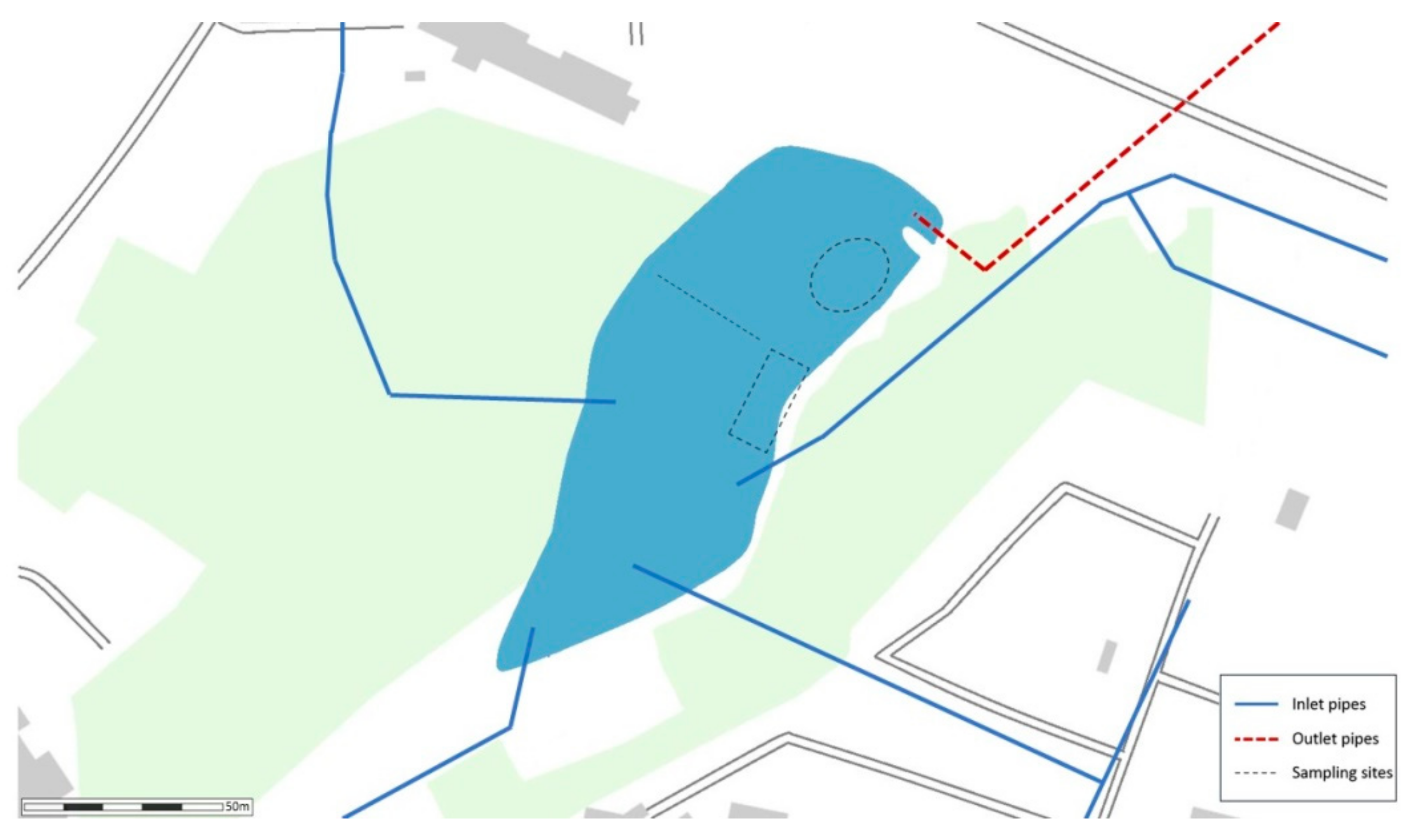A horizontally rectangular map with a predominantly white background. Central to the map is a large, muted pastel light green area, indicative of grassy land, with a rectangular teal shape symbolizing water. Towards the lower left corner, a light gray banner with two dark gray lines suggests a legend, though the text is unreadable. The lower right corner features a black-outlined legend box, detailing the map's elements: thin blue lines indicate inlet pipes, dotted red lines signify outlet pipes, and faint gray dotted lines mark sampling sites. Several blue and red lines extend from various directions towards the teal water area, possibly marking railroad tracks or pathways. Additionally, a scale at the bottom denotes a distance of 50 meters. Scattered across the map are small, illegible squares, likely identifying specific features.